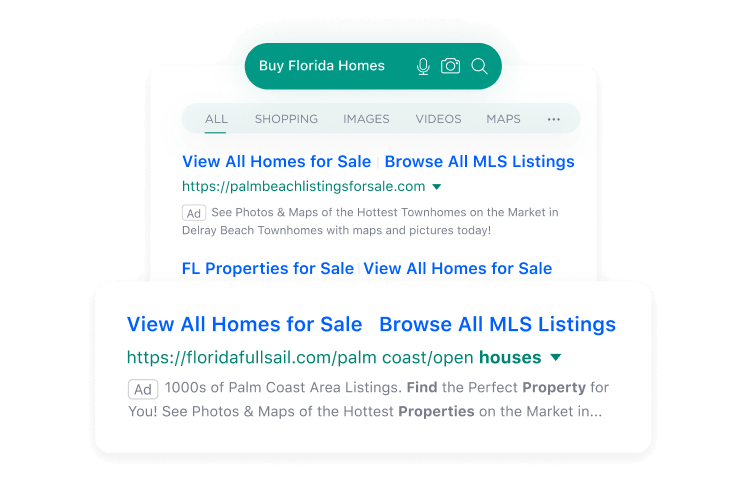At the top of the image, there's a dark green oblong box featuring the text "Buy Florida Homes." The box is accompanied by three icons: a microphone, an image icon, and a search icon. Below this, a gray menu bar presents options labeled "All," "Shopping," "Images," "Videos," and "Maps," followed by an ellipsis. 

Further down in blue text, it reads, "View All Homes for Sale, Browse All MLS Listings." Underneath, a green URL is displayed: "https://palmbeachlistingforsale.com." Following this, gray text states, "See Photos and Maps of the Hottest Townhomes on the Market and Delray Beach Townhomes with Maps and Pictures Today." 

Below this in blue text again, it says, "Florida Properties for Sale, View All Homes for Sale." A smaller box beneath this repeats in blue, "View All Homes for Sale, Browse All MLS Listings," followed by another green URL: "https://floridaforsale.com/Palm-Coast/Open-Houses." It concludes with the gray text, "Thousands of Palm Coast Area Listings."